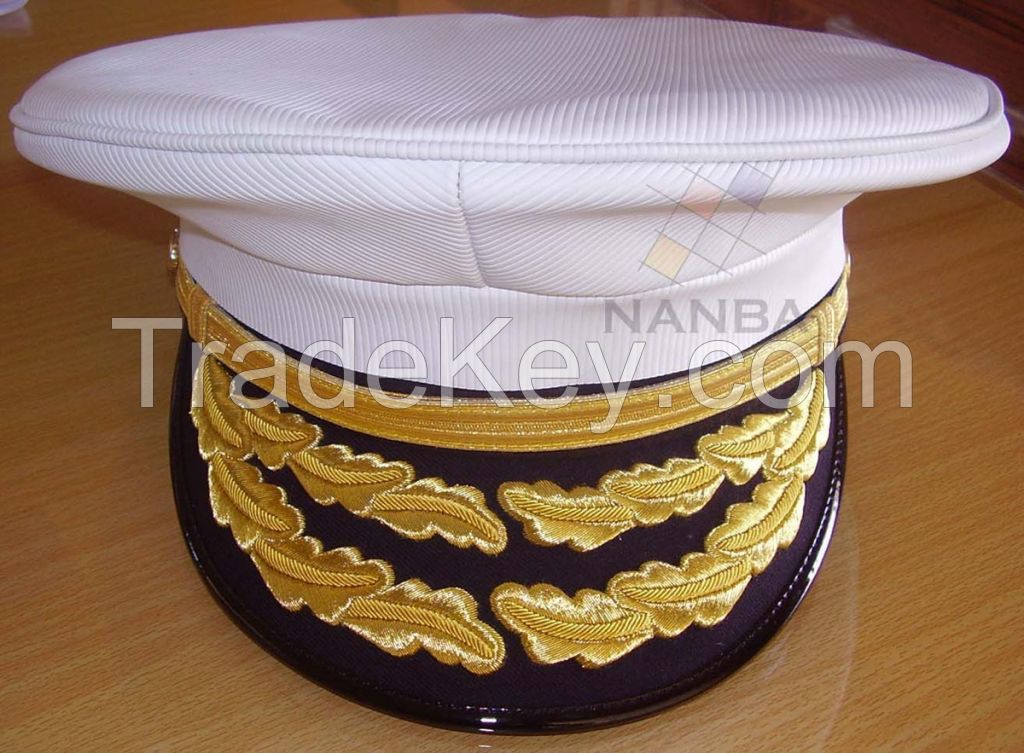The close-up image features an elaborate military-style hat resting on a smooth, highly reflective wood surface. The hat is predominantly white, with a flat-topped fabric crown that extends outwardly. Its brim is richly adorned with intricate gold embellishments, prominently featuring leaf embroidery on a black background, and secured by a gold band with a knob on the left-hand side. The hat also includes transparent text overlays, with "TradeKey.com" displayed underneath "NANBA" across the upper portion of the white fabric, along with a mesh-like logo in a small section above them. The overall style of the hat resembles that of a Navy officer, although not of a commonly recognized design.